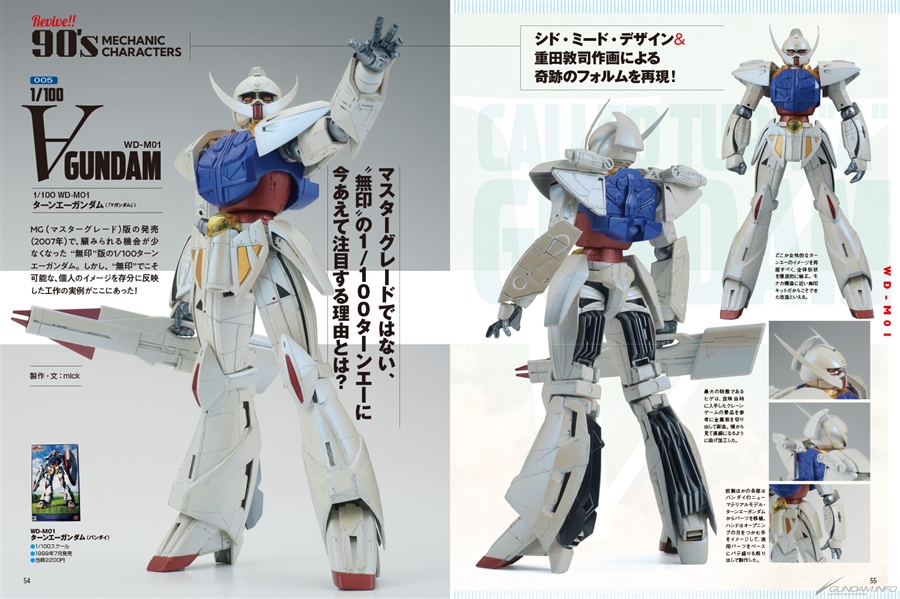This detailed image is a promotional spread, potentially from a magazine or catalog, showcasing the action figure or character design of a V Gundam, designated as WD-MO1. The image presents the Gundam in various poses and angles, accompanied by descriptive text primarily in Japanese. The caption "Revive 90s Mechanic Characters!!" is prominently displayed at the top left in red, followed by "005" and "1-100" in black, indicating its place in a series.

The central figure of the Gundam is predominantly white, accented with red on its knee pads and the tips of its high-heeled feet. It features a blue chest plate with red underneath and a gold belt buckle. The Gundam's right hand holds a weapon that appears to be a white, red-tipped sword, while its left hand is raised with an open grasp.

The helmet is distinct with white horns or tusks protruding from each side, resembling a Viking helmet. Additional details include gray hands and beige armor on the back, resembling a rectangular shape with pointed ends. The back of the legs reveals some grey metallic components, emphasizing its mechanical design.

Smaller images within the spread provide close-up views of the head, back, arms, and legs, illustrating the intricate details and articulation of the model. Text in Japanese accompanies these images, providing further context and specifications. The background alternates between gray and white, reinforcing the high-quality and professional presentation typical of a magazine or catalog layout.